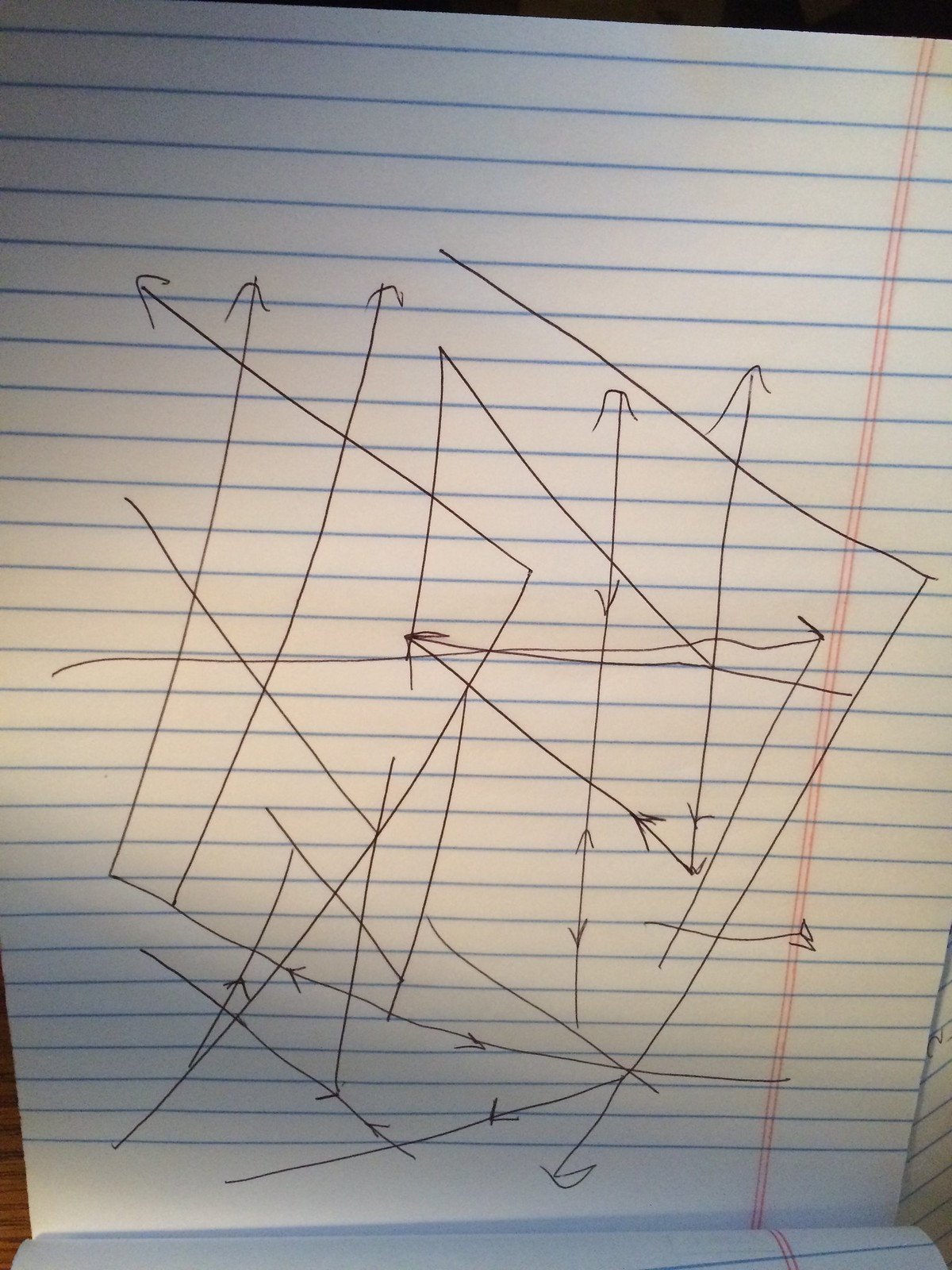The image depicts an upside-down legal pad of paper, with the top sheet flipped over such that the left-hand margin appears on the right. The paper is standard lined, featuring two distinct red vertical margins and blue horizontal lines against a white background. The main focus is a series of black pen-drawn arrows crisscrossing the page in various directions. These arrows form a chaotic, almost square-like pattern, with some creating 90-degree angles, pointing upwards, downwards, and sideways. Notably, there are no written words on the page, just an intricate arrangement of multi-directional arrows that collectively give a sense of dynamic movement.